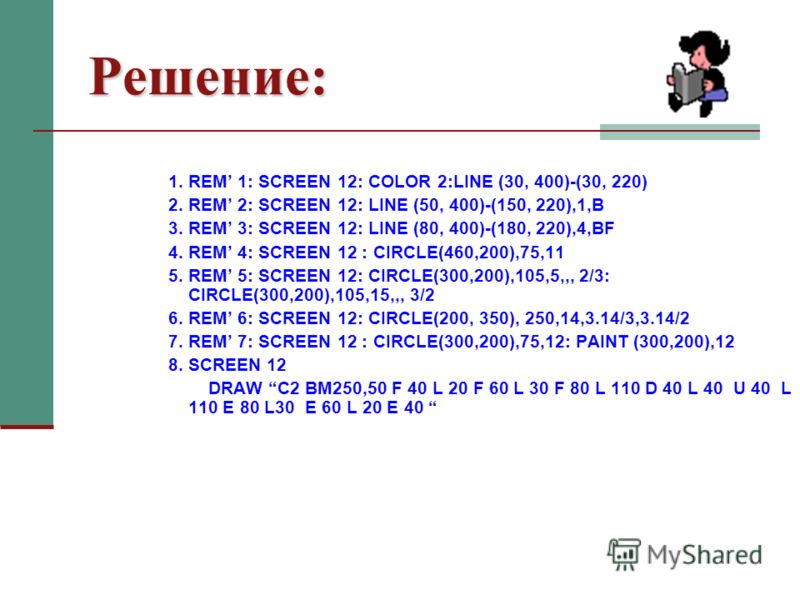The image is a screenshot of a white-background webpage. A dark green rectangular border runs vertically along the left side. In the upper left corner, a title in dark reddish-brown letters reads "P.E. III E.H.N.E." On the opposite side, the upper right corner features a cartoon drawing of a girl with black hair sitting and reading a gray book. Beneath these elements is a horizontal dark reddish-brown line that spans the page, partially highlighted in green on the right side.

Below the line, there are eight numbered lines of text, each starting with "R.E.M." followed by instructions, likely script code:
1. "R.E.M. 1; SCREEN 12; COLOR 2; LINE (30, 400) - (30, 220)"
2. "R.E.M. 2; SCREEN 12; LINE (50, 400) - (150, 220), 1, B"
3. "R.E.M. 3; SCREEN 12; LINE (80, 400) - (180, 220), 4, B, F"
4. "R.E.M. 4; SCREEN 12; CIRCLE (460, 200), 75, 11"
5. "R.E.M. 5; SCREEN 12; CIRCLE (300, 200), 105, 5, , , 2/3; CIRCLE (300, 200), 105, 15, , , 3/2"
6. "R.E.M. 6; SCREEN 12; CIRCLE (200, 350), 250, 14, 3.14/3, 3.14/2"
7. "R.E.M. 7; SCREEN 12; CIRCLE (300, 200), 75, 12; PAINT (300, 200), 12"
8. "SCREEN 12; 1-10-E; 80-L; 30-E, 60-L, 20-E, 40"

In the lower right hand corner, an image of a small computer is displayed, with the text "my shared" right-aligned in gray letters.